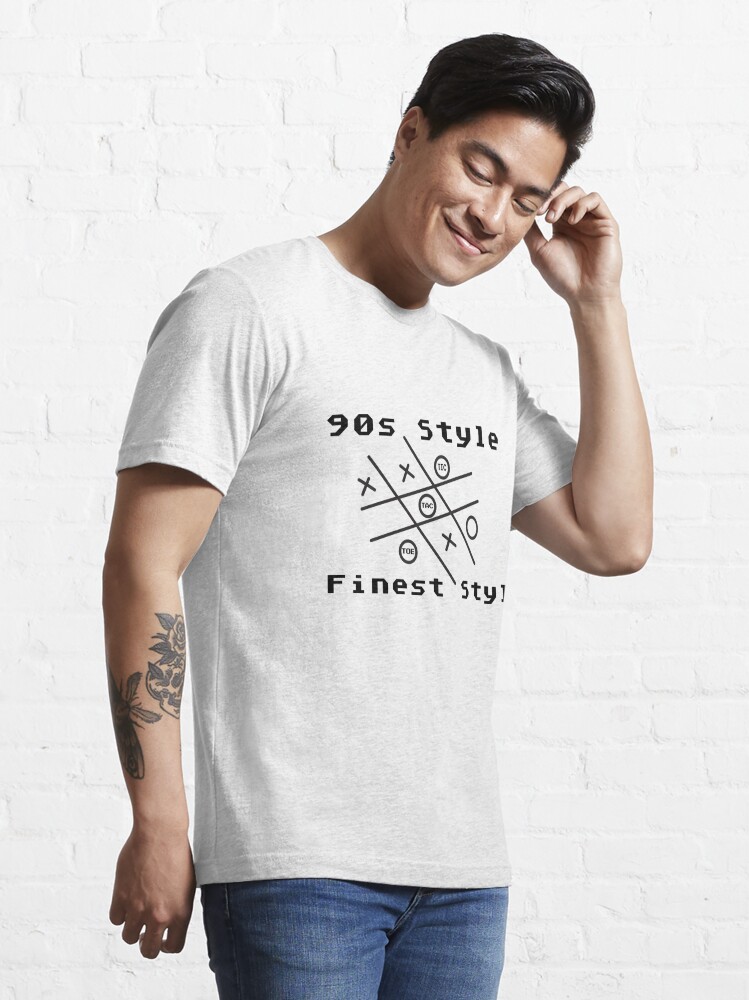The image features an Asian man standing against a solid white brick wall. He has short, styled black hair combed to one side and wears an off-white t-shirt decorated with a graphic of a tic-tac-toe game. The shirt has the phrases "90's style" above the graphic and "finest style" below it, written in a playful, almost Pac-Man style font with mostly lowercase letters. The tic-tac-toe board shows three X's and four O's, with three O's aligned diagonally to form a winning line. The man is wearing blue jeans and has a thoughtful expression, with his left hand lifted near his face and his right arm hanging by his side. His right forearm is adorned with a detailed black-and-white tattoo of a flower bush, exhibiting a fine line style.